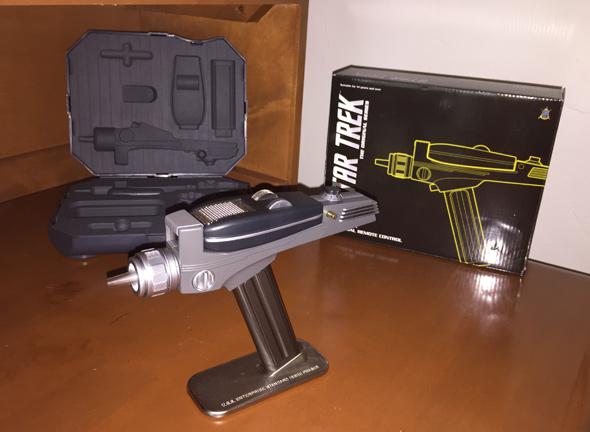The image displays a meticulously crafted toy phaser from the original Star Trek series, prominently centered and positioned diagonally on a glossy brown floor. This detailed replica is predominantly grey, with black and silvery-dark grey accents, and is oriented to the left side of the image. Behind the phaser, an open grey suitcase-like carrying case reveals precisely cut foam slots designed to house the phaser's various components, highlighting the realistic, assemble-it-yourself nature of the toy. To the right, a black box, clearly distinguishable by its vertical white "Star Trek" lettering and yellow phaser image, stands against a white wall background. The setting effectively captures the authentic and nostalgic essence of Star Trek merchandise.